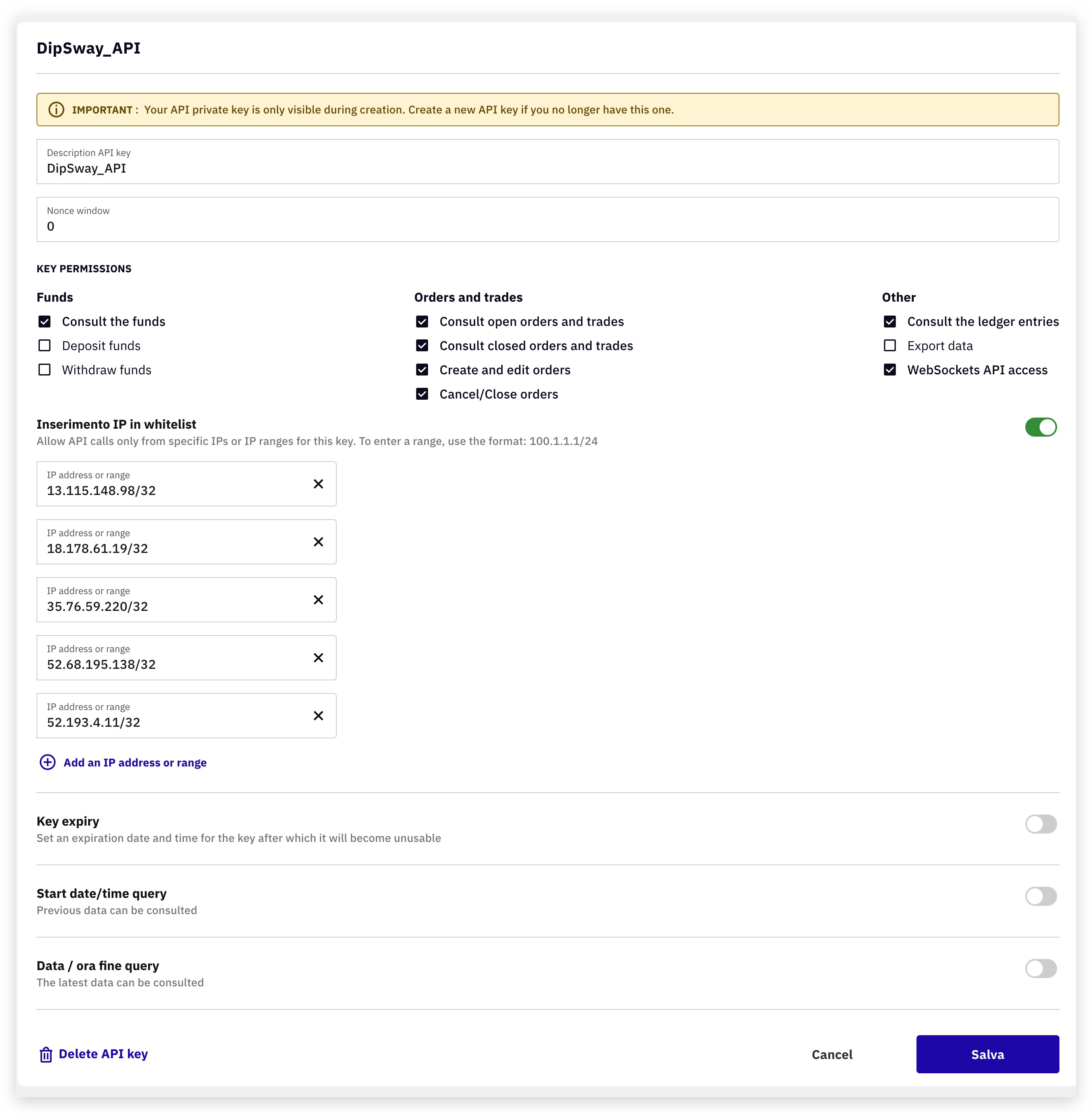This image is a screenshot of a website, featuring a predominantly white background with black text, encased in a gray border that gives it a square appearance. 

### Header
Located at the top-left corner, the header reads "dip sway_api" and includes a prominent yellow notification box. This box contains the message: "Important: Your API private key is only visible during creation. Create a new API key if you no longer have this one."

### API Key Sections
Beneath this, there is a white text box that again displays "dip sway API." Adjacent to this is another empty white box.

### Key Permissions
Further down, under the section titled "Key Permissions", various permissions are indicated:
1. **Funds:**
   - Consult the funds (checkbox selected).
2. **Orders and Trade:**
   - Consult open orders and trades (checkbox selected).
   - Consult closed orders and trades (checkbox selected).
   - Create and edit orders (checkbox selected).
   - Cancel close orders (checkbox selected).
3. **Other:**
   - Consult the ledger entries (checkbox selected).
   - WebSockets API access (checkbox selected).

### IP Whitelist
Below the permissions section, there is a portion titled "IP Whitelist." This section includes input boxes for varying IP addresses or ranges, which are populated with numerous numbers.

### Footer
At the bottom-right corner of the screenshot, there are two buttons. "Cancel" is displayed in a standard format, while "Salva" is highlighted in a blue box, indicating it is the button for saving changes.

This detailed caption aims to comprehensively describe the elements and layout of the screenshot.